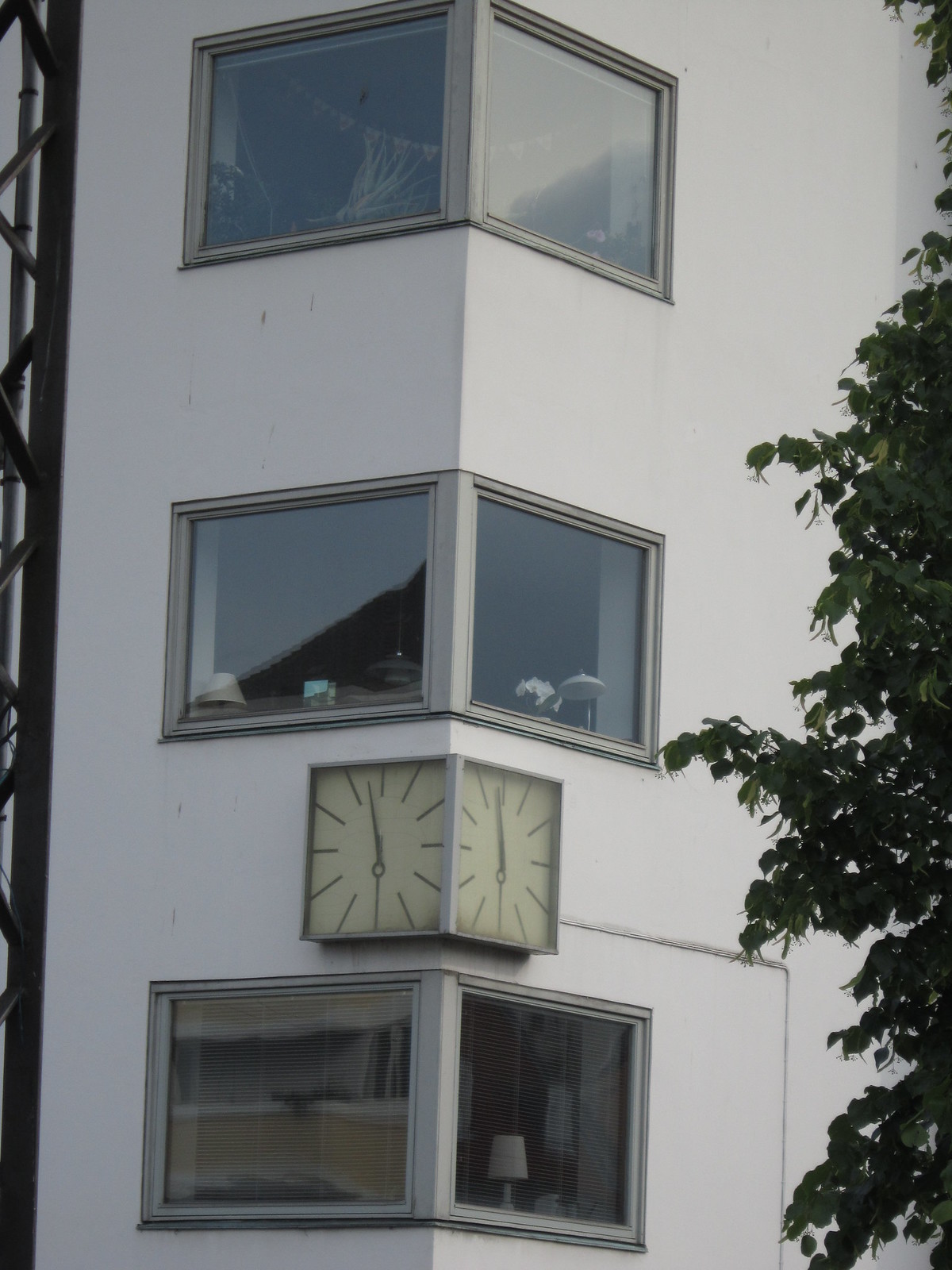The color snapshot showcases the corner of a three-story white building featuring a distinctive V-shaped configuration created by large, abutting corner windows on each floor. The windows, which straddle the corner of the building, reveal various items inside, including lamps and a hat. Between the first and second floors, there are dual clock faces aligned in a V-formation, mirroring the angle of the windows. These clocks, devoid of numbers, appear to indicate a time close to 5:57 PM. The facade is flanked by a large tree with abundant ivy-like leaves on the right side, while an unidentified black metal structure, possibly a fire escape or scaffolding, ascends the left side.